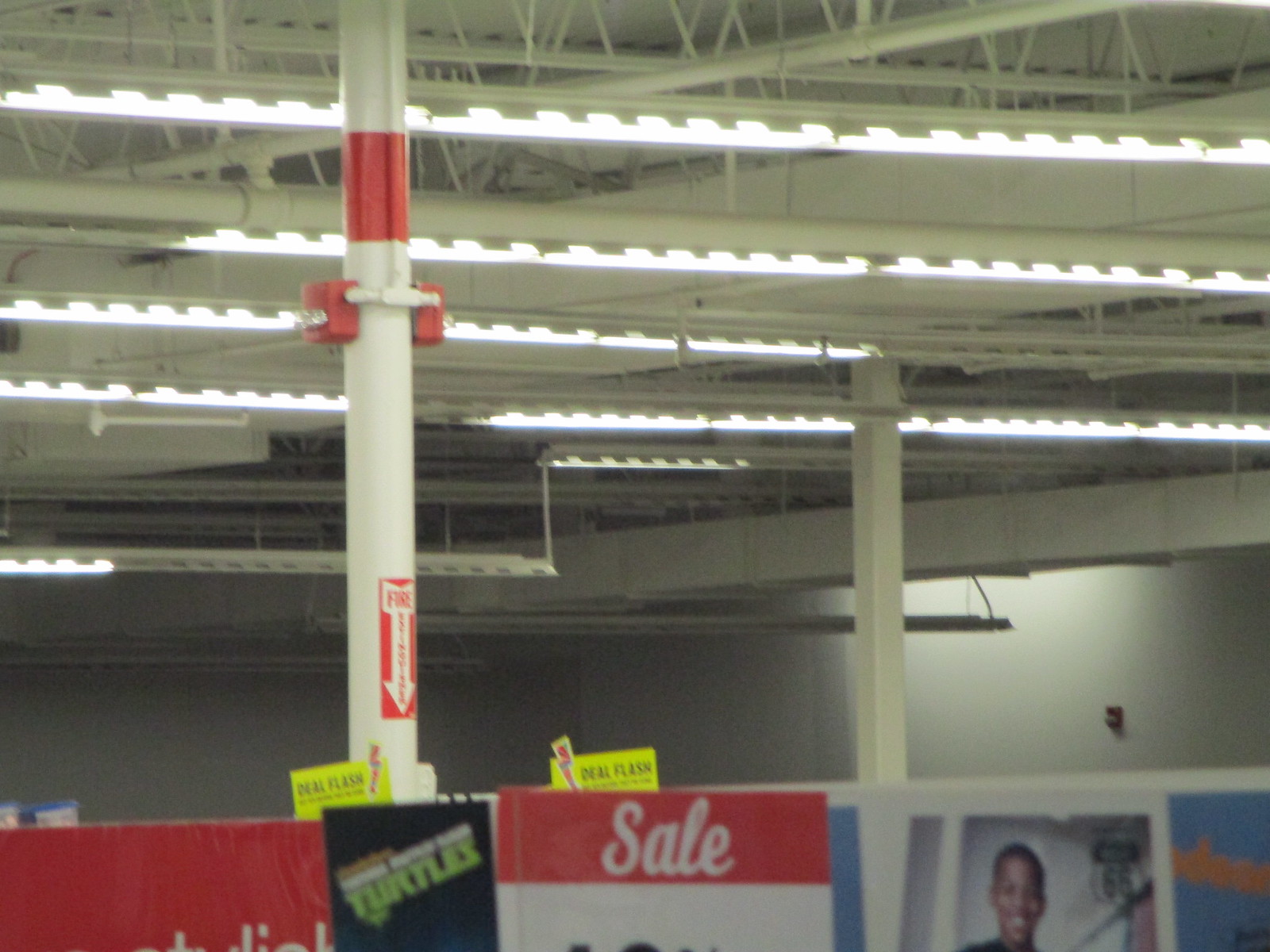The image depicts the top section of a store, highlighting its ceiling and signage. At the bottom of the image, a series of partially visible signs can be seen. The sign on the far left is red. Adjacent to it is a black square sign with the green word "turtles" at the bottom. To its right, there is a sign that is half red and half white; the top portion, in red, displays the word "sale" in white cursive text, while the lower portion is plain white. Next, an image of a child is visible, facing forward. Further to the right, a blue sign with some orange text is partially visible. In the area above, a vertical white pole with a red stripe and the word "fire" written near the bottom, accompanied by a fire alarm, is noticeable. The walls in the background are gray. The ceiling dominates the majority of the image, displaying an intricate network of light gray beams and pipes, interspersed with several white lights running along the piping.